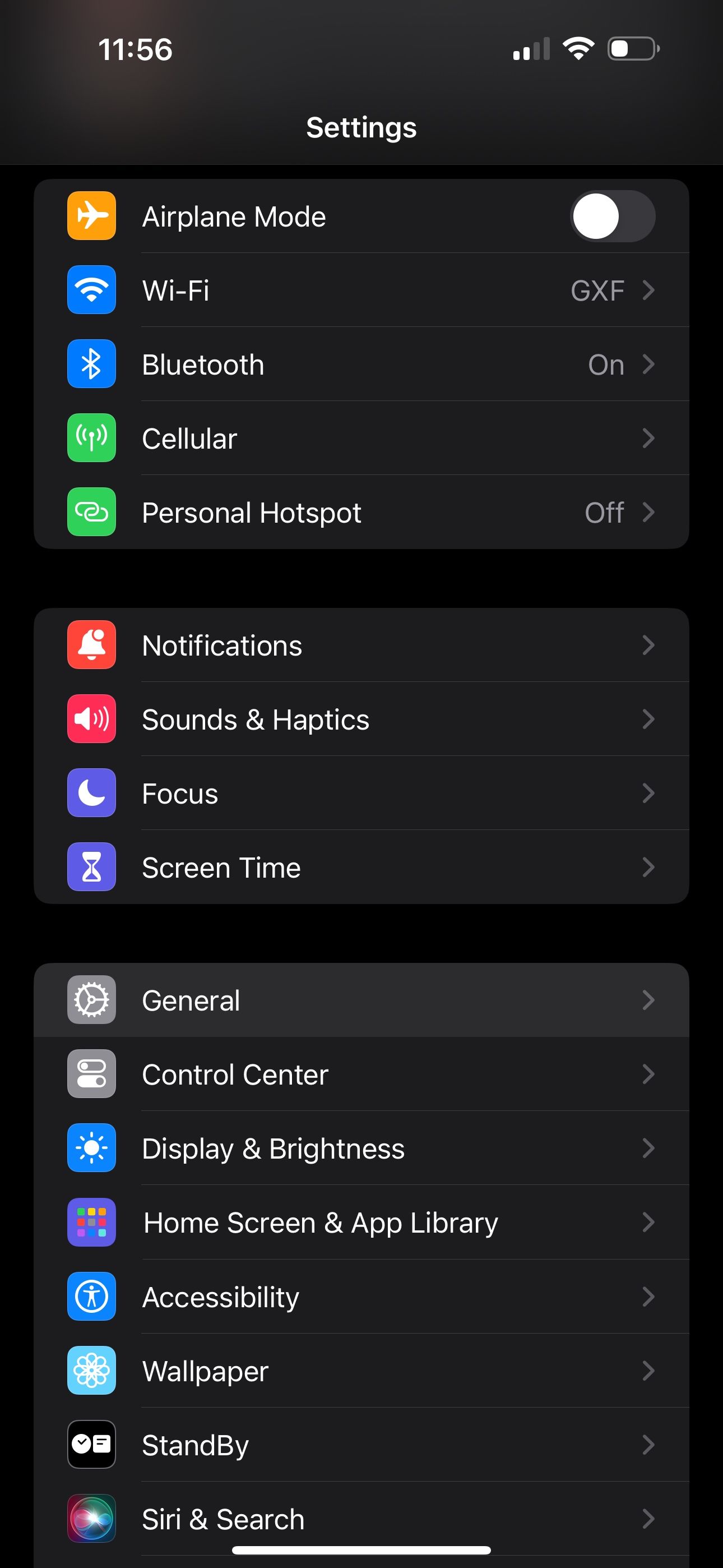The image depicts a smartphone's screen displaying its "Settings" menu. 

At the very top of the screen, the status bar includes detailed indicators: the time (11:56) on the left-hand side, and icons for signal strength, Wi-Fi connectivity, and battery life on the right-hand side. 

Directly below the status bar, against a dark grey background, the word "Settings" is prominently displayed in white, centered at the top of the screen.

Beneath the title, a structured interface presents various settings options:

- **Airplane Mode**: Indicated by an orange button with an airplane icon, which appears to be enabled.
- **Wi-Fi**: Set to "GXF."
- **Bluetooth**: Currently turned on.
- **Cellular**: Marked by a green button and an expandable right-arrow icon.
- **Personal Hotspot**: Displayed with a green icon, which is currently off.

These primary settings are followed by a middle section containing categories:

- **Notifications**
- **Sounds & Haptics**
- **Focus**
- **Screen Time**

Lastly, the bottom section features additional settings options:

- **General**: Highlighted as the currently selected option.
- **Control Center**
- **Display & Brightness**
- **Home Screen & App Library**
- **Accessibility**
- **Wallpaper**
- **Standby**
- **Siri & Search**

Each section is systematically organized with icons and labels, providing a comprehensive overview of the smartphone's configuration options.